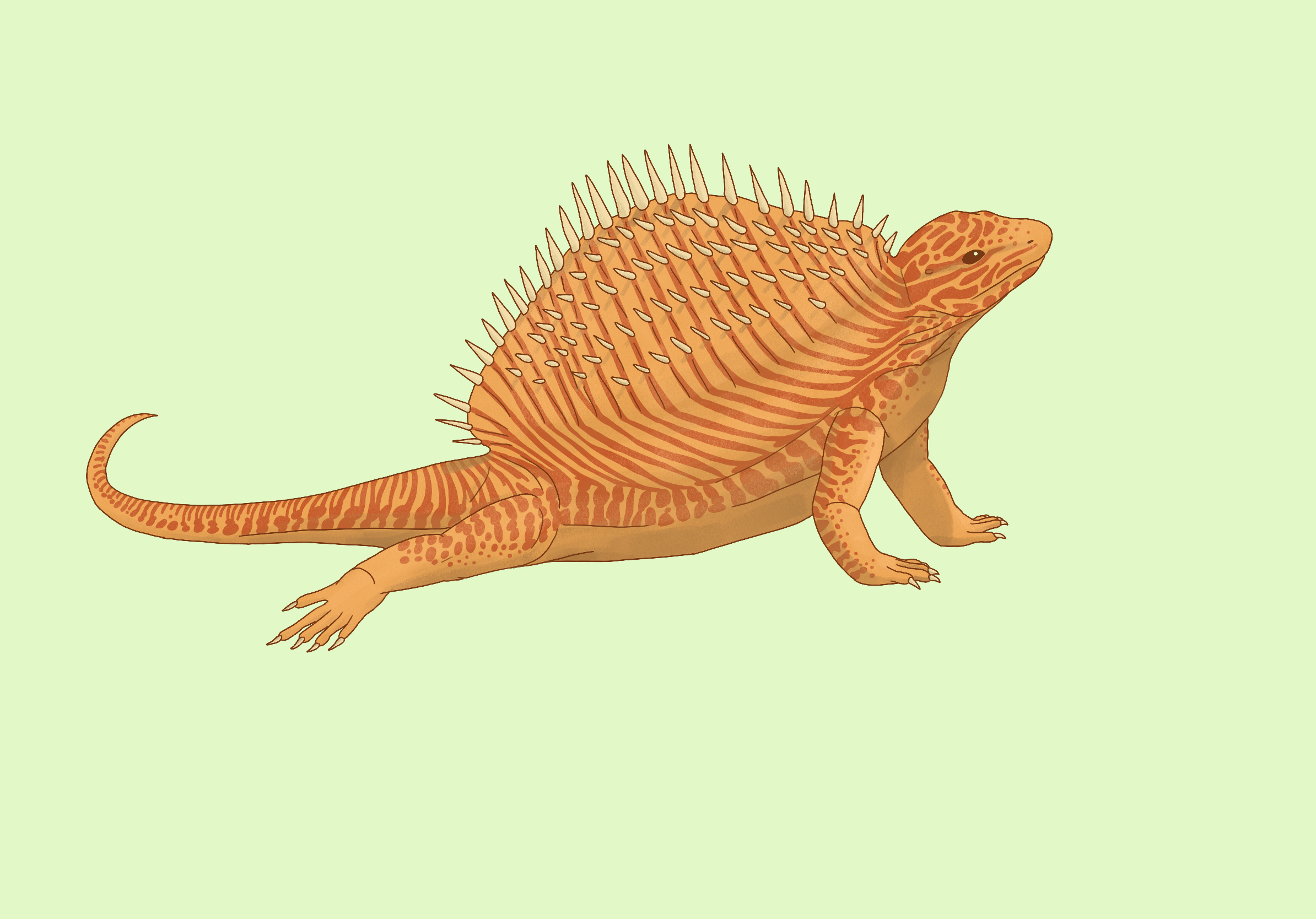This illustration features a distinctive reptilian creature prominently centered against a soft pastel green background. The drawing is inked with dark brown lines, highlighting the detailed anatomy of the lizard-like creature. The lizard itself has a predominantly beige coloration, accented with an array of orange and darker brown stripes along its top. The creature's head, which is turned towards the upper left corner of the image, features a prominently visible white eye with a noticeable dark pupil.

One of the most striking features of the lizard is a large, humped shell on its back. This shell is adorned with alternating red and beige stripes and is covered in numerous small beige spikes, giving it a formidable appearance. The lizard is depicted standing on its two front legs, with both rear legs appearing to drag behind it, visible is only one rear leg. Its long tail is curled and extends to the left side of the image.

The lower part of the lizard’s body, including its belly, is monocolored in beige, providing a sharp contrast to the more intricately patterned and colored upper part. The creature's overall presentation is set against a large square gray background, which further emphasizes the unique details and colors of the lizard, making the illustration both detailed and visually engaging.